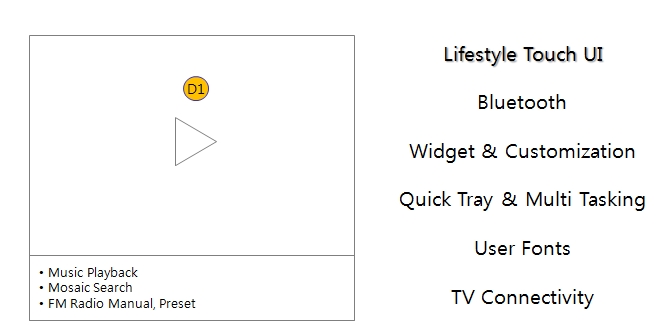The image features a simple diagram on the left side, consisting of a black-outlined rectangle on a white background. Inside this rectangle, there's a right-pointing triangle resembling a play button. Above this triangle sits a small, yellow circle with the text "D1" inside it. Below this diagram, a vertical list in black text reads: "Music Playback," "Mosaic Search," and "FM Radio Manual, Preset." To the right of the diagram, another vertical list in black text showcases various features: "Lifestyle," "Touch UI," "Bluetooth," "Widget and Customization," "Quick Tray," "Multitasking," "User Fonts," and "TV Connectivity." The overall design is basic and clearly organized.